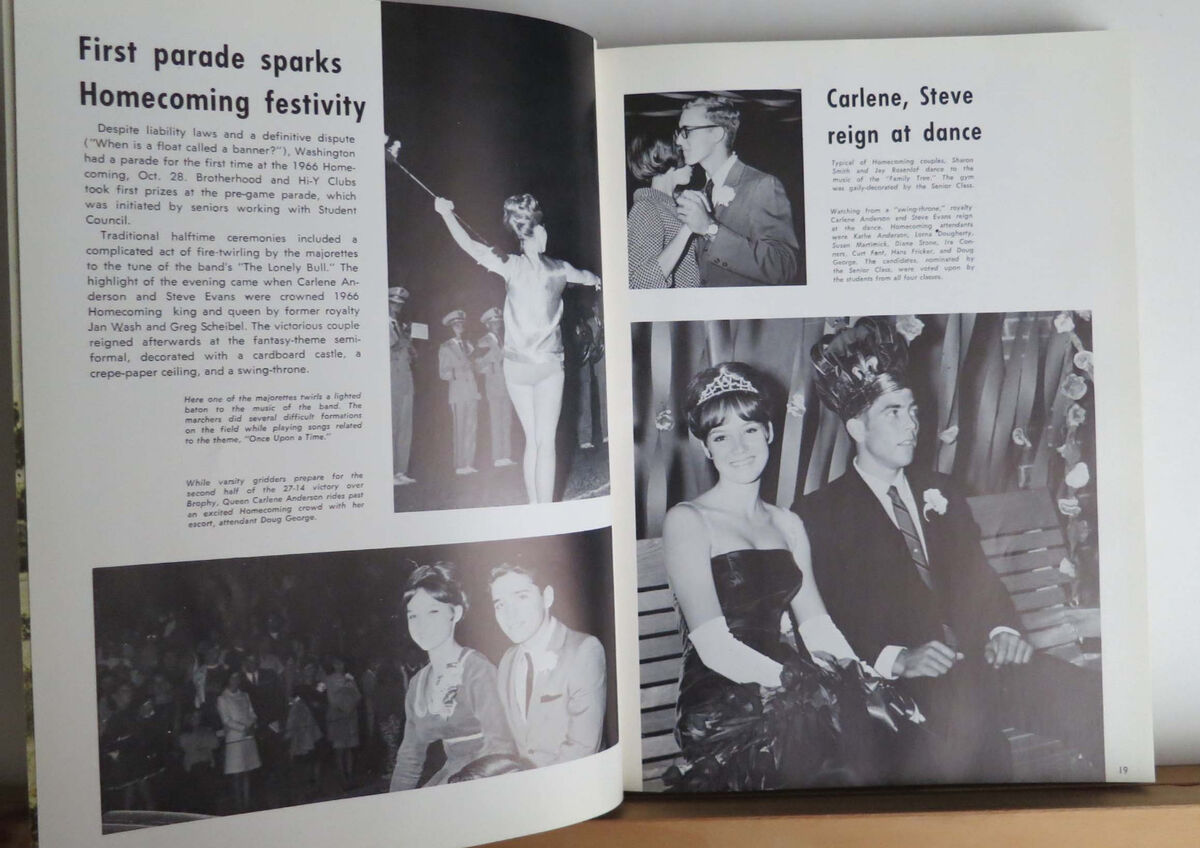The black-and-white image appears to be an open two-page spread from an old yearbook, placed on a brown surface with a white wall in the background. On the left page, the header "First Parade Sparks Homecoming Festivity" is seen, accompanied by a couple of paragraphs underneath. The top of the page features a photograph that appears to capture a marching band in the background, with a young man and woman sitting together while other people stand in the distance.

The right page presents several smaller photographs and text captions. In the upper section, there is an image of a man and woman dancing, with the caption "Charlene, Steve, Rain and Dance" in black letters. At the bottom of the right page, there is a photograph of a young woman in a dark-colored dress sitting beside a young man in a dark suit on a bench, both likely being honored as the homecoming queen and king. The entire spread suggests a celebratory event surrounding a homecoming parade and dance, capturing moments of proud student achievements and communal festivities.